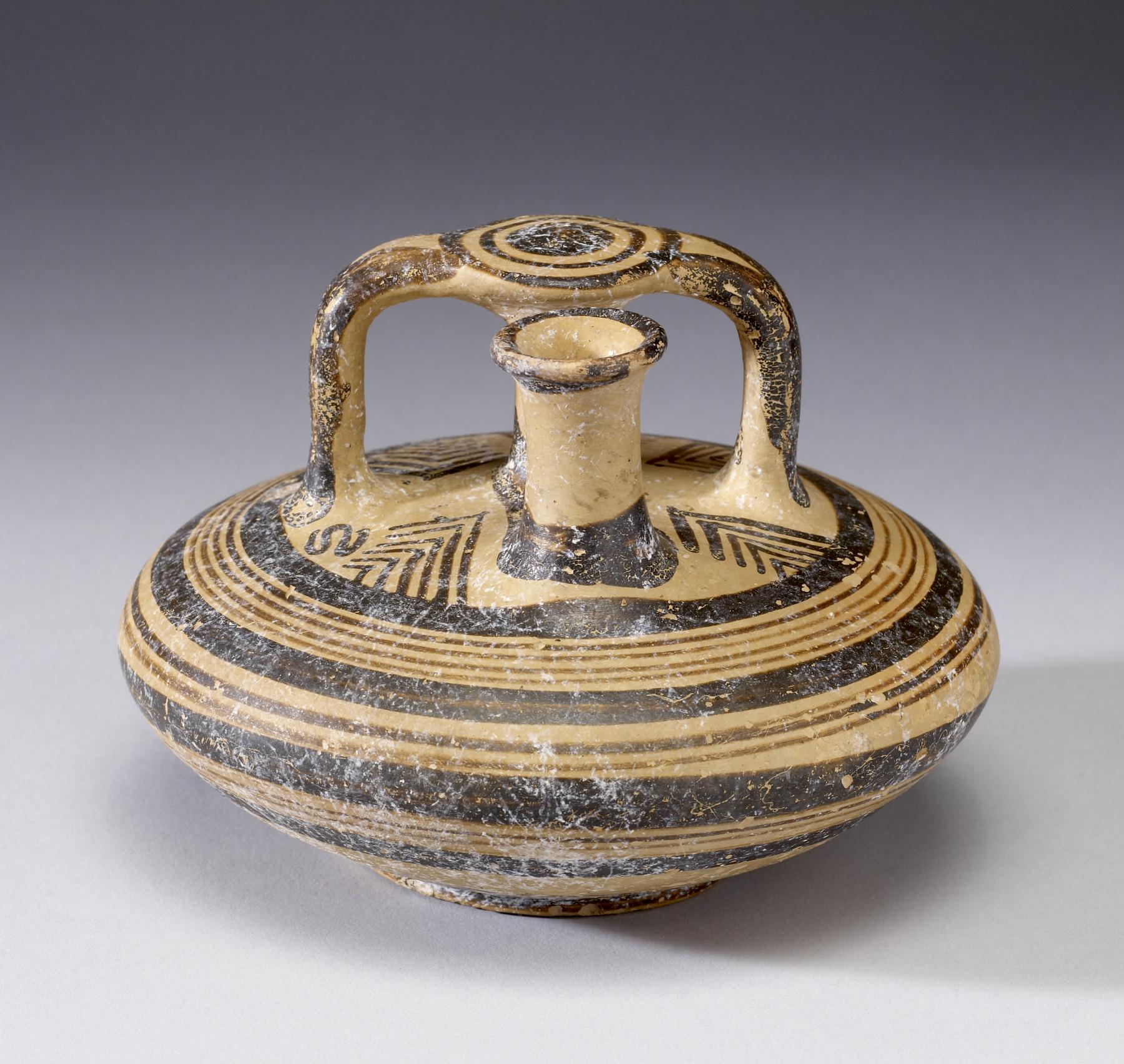The image depicts an ancient clay pot, likely an artifact preserved in a museum, placed on a plain white tabletop to emphasize its features. This weathered pot, which appears to be of considerable age reminiscent of Aztec pottery, has a distinctive shape: it starts narrow at the base, expands broadly towards the middle, and then tapers back in at the top, culminating in a small, tubular opening about the width of a Gatorade bottle cap. This opening, which extends approximately two inches from the main body, is likely designed for pouring substances like oil or water, which the pot may have been used to transport. Attached behind this spout is a handle that facilitates lifting and pouring. The pot is adorned with intricate dark brown patterns, featuring lines, circles, and what appear to be snake motifs, all contributing to its ancient and possibly ritualistic aesthetic. Despite the beauty of these markings, the surface shows signs of wear, indicating its long history and usage.